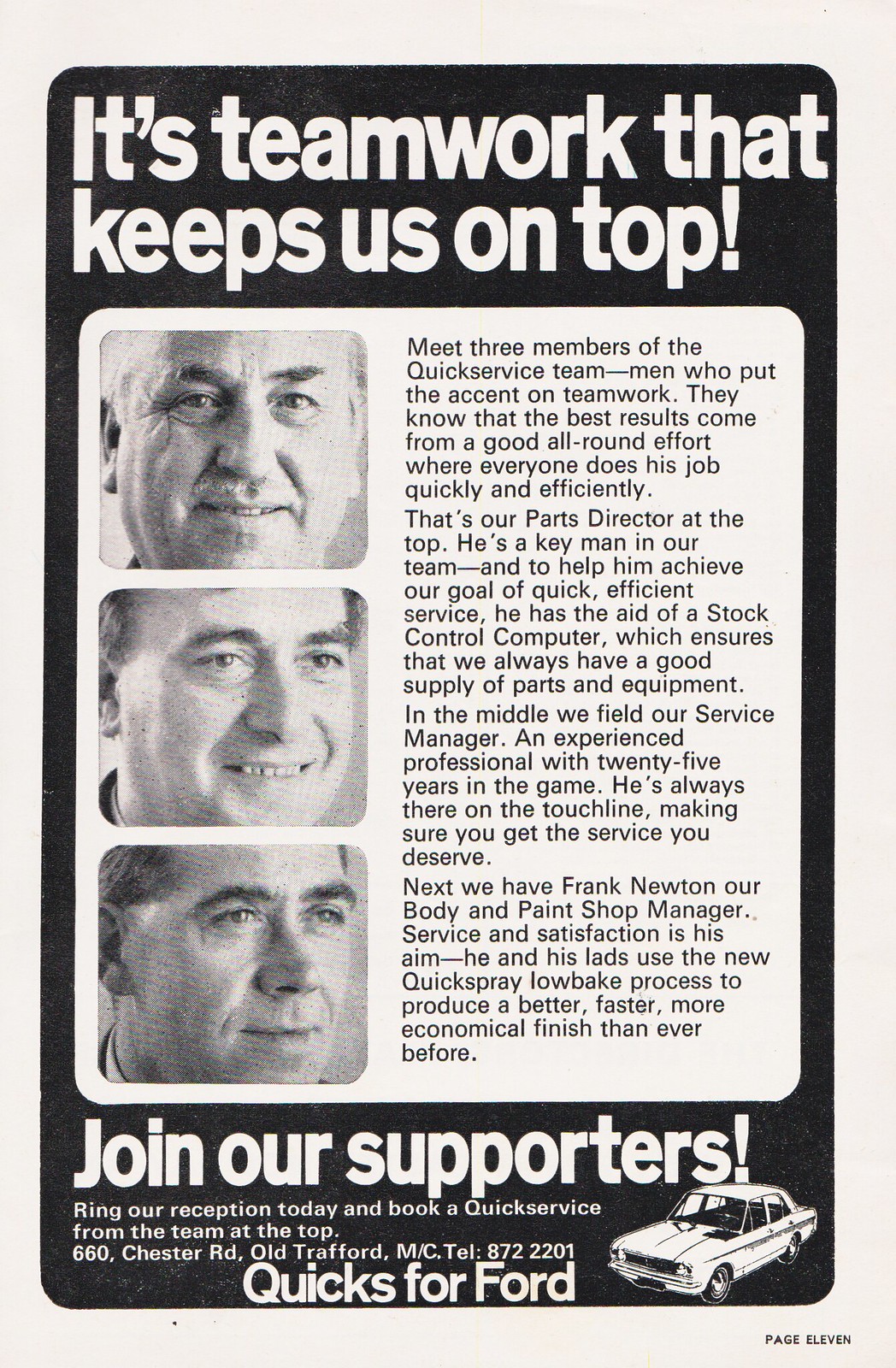The image is a black-and-white advertisement, likely from a magazine, centered on teamwork within an automotive dealership's quick service team. The photo is set against a light gray background, featuring a black box with white text that reads, "It's teamwork that keeps us on top." Inside this box, on the left side, are black-and-white headshots of three Caucasian men, stacked vertically, each representing a key member of the team.

The man at the top is identified as the parts director, an essential figure supported by a stock control computer to ensure a steady supply of parts and equipment. Below him is the service manager, a seasoned professional with 25 years of experience, always present to ensure top-notch service. The third member’s role is not explicitly detailed but they are also integral to the team's success.

On the right side of the black box, there are three detailed paragraphs of black text that emphasize the importance of teamwork in achieving efficient and effective service, where everyone's quick and proficient efforts contribute to the best outcomes. Below, the text reads, "Join our supporters. Ring our reception today and book a quick service from the team at the top," along with the contact details: "660 Chesa Road, Old Trafford, M/C, tel: 872-2201."

The bottom of the image features a small drawing of a car and the page number "11," indicating its place within the magazine.